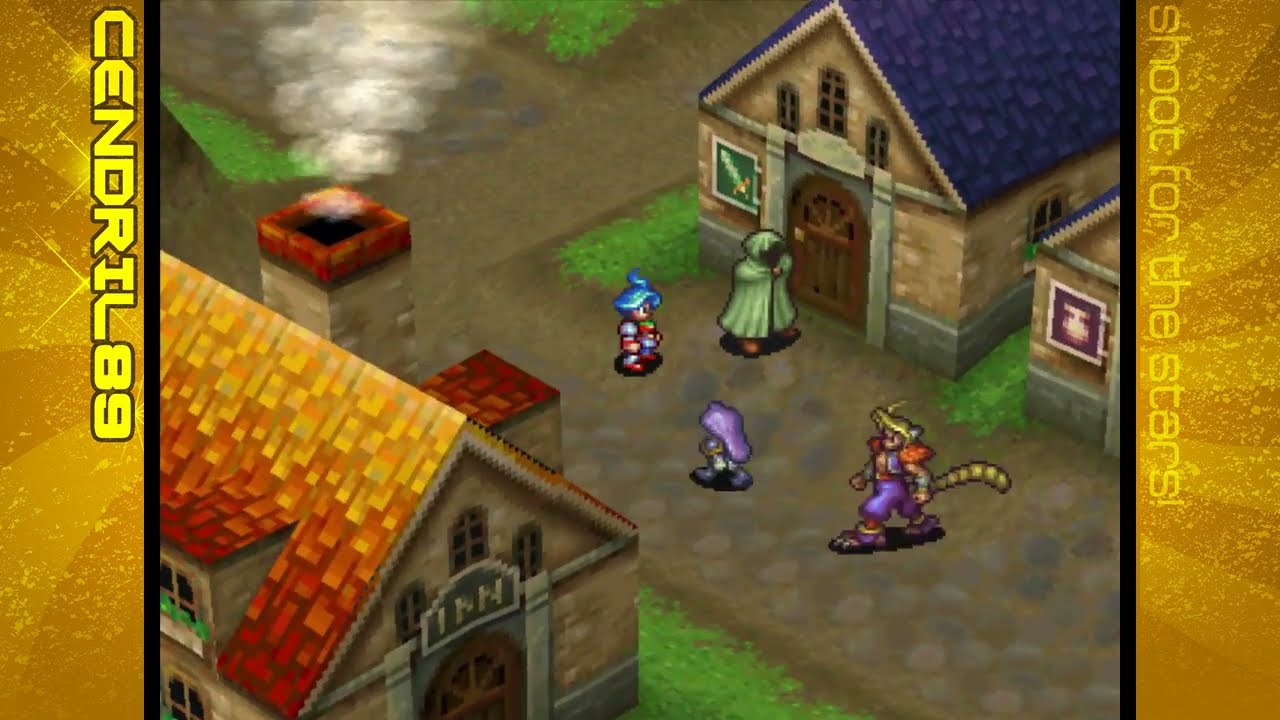This screenshot from a video game exhibits a richly detailed fantasy scene, framed by ornate gold borders with alternating sunbeam patterns. The left border features vertically oriented text that reads "Central 89," suggesting a potential reference to either a game title or character handle, while the right border displays the motivational phrase "Shoot for the Stars." Central to the image is a bustling town street flanked by various buildings. On the bottom left, there is a two-story inn with stone walls and an orange-red sloped roof, emitting smoke from a chimney. Adjacent buildings feature icons for weapons and potions, likely indicating an armory and an apothecary.

The scene is populated by four distinctive characters: a cloaked figure in a light green cloak, a smaller character with blue hair wearing armor, another armored character with purple hair, and a humanoid figure with blonde hair and a tail, clad in purple shorts or pants and adorned with red shoulder pads. These characters stand amidst patches of grass interspersed between the structures, adding a layer of interactivity and liveliness to the quaint, medieval town ambiance.